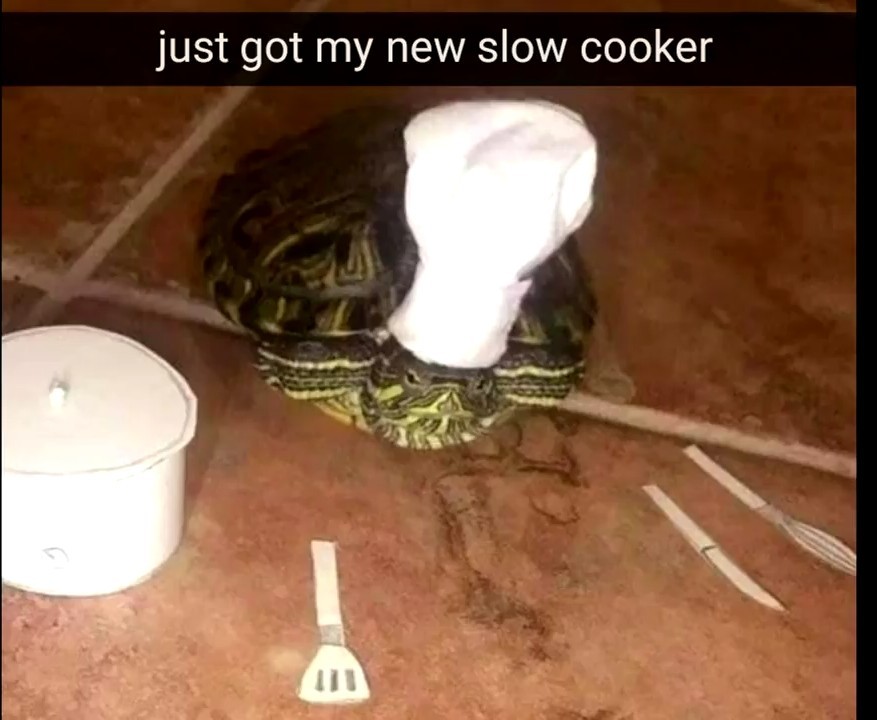This image presents a comedic scene featuring a green turtle adorned with a traditional white chef’s hat, lying on a brown and red tiled floor. The background is dark, likely emulating a kitchen counter. A black bar with white text at the top humorously states, "Just got my new slow cooker," playing on the turtle's slow movement. 

The turtle, predominantly green with dark and light green stripes, is centrally positioned with its head partially emerging from its shell while its legs are mostly retracted. Surrounding the turtle is an array of small, cut-out kitchen utensils that appear hand-drawn on white paper. To the left of the turtle sits a tiny white pot, and in front of it are a spatula, a knife, and a whisk. These utensils, along with the pot, feature simple white designs with shading to mimic depth, complementing the whimsical theme of the image. The elements collectively suggest a light-hearted and imaginative take on kitchen-themed humor.